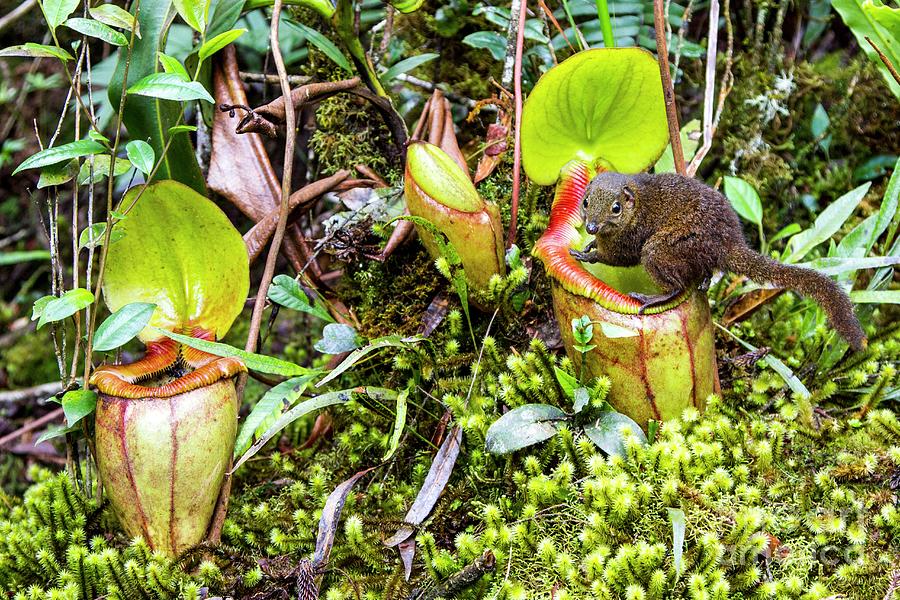In this detailed photo, a brown, furry squirrel stands poised on a green and red pitcher plant in the midst of a lush garden. The squirrel, with its long tail and prominent paws gripping the rim of the carnivorous plant's pitcher, gazes directly at the camera. The garden features two prominent pitcher plants with large stems and leaves, one in the left-hand corner and another in the right middle of the image. The pitchers, characterized by their green hue with red accents, are surrounded by an array of small, spiky plants protruding from the ground. The backdrop is a rich tapestry of various shades of greenery, consisting of small plants, leaves, grass, and twigs, blending seamlessly into the forest beyond. The image, taken outdoors, showcases a myriad of colors including light green, brown, black, gray, yellow, and off-color blue, capturing the vibrant and diverse ecosystem within the garden.